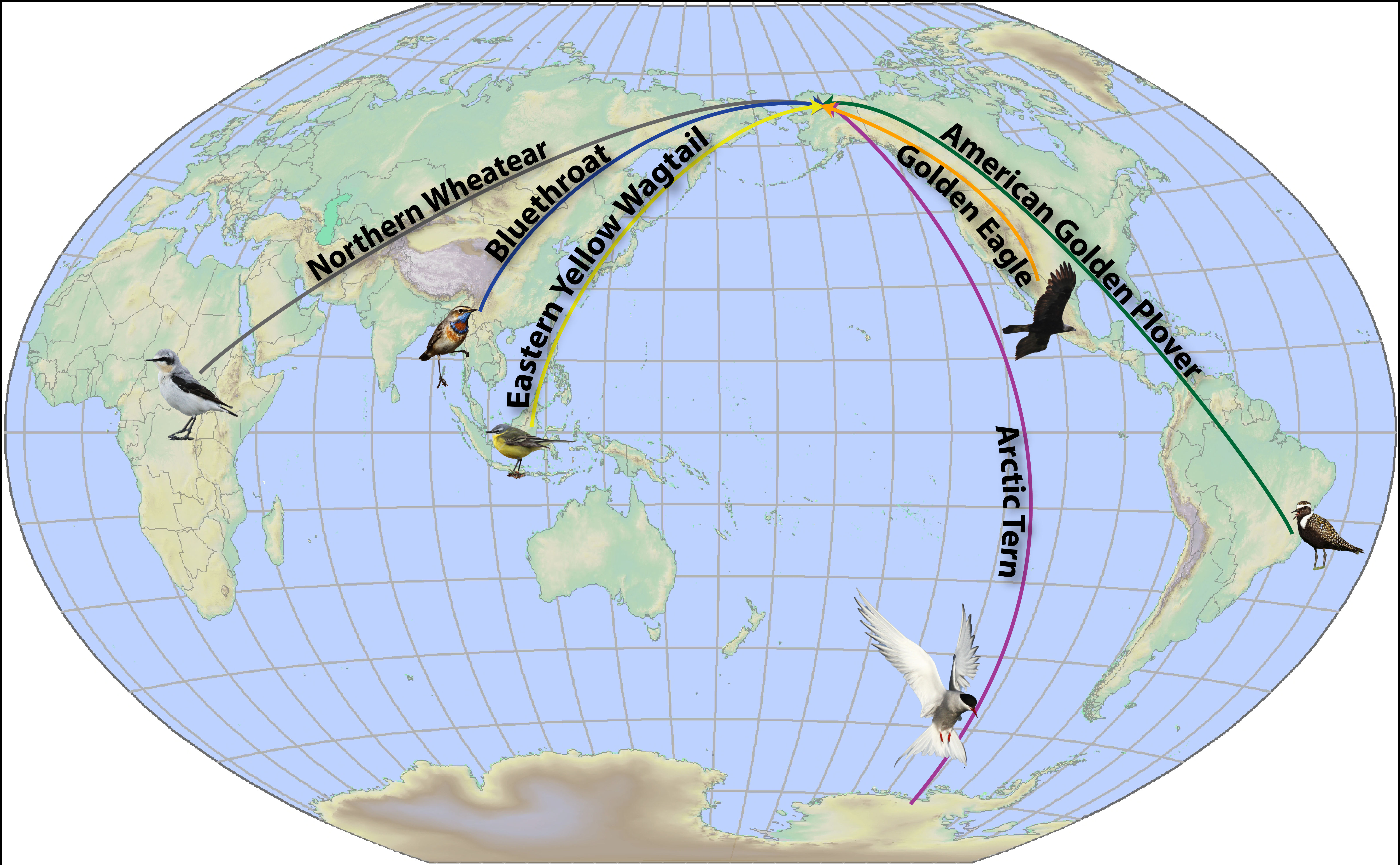This image features a stretched-out, semi-spherical representation of the globe showcasing various continental regions and the birds native to them. Starting from the left, a gray line points to Africa, labeling the Northern Wheatear, a black and white bird. Moving right to Asia, a blue line identifies the Blue Throat, a bird adorned with brown, orange, red, and blue hues. Adjacent is the Eastern Yellow Wagtail, marked by a yellow line, a gray bird with a vibrant yellow chest and stomach. Continuing right, a pinkish-purple line marks the Arctic Tern, depicted in white with a gray body, black head, and red beak, flying towards the Arctic. Over North America, Central American area, a golden line highlights the majestic Golden Eagle, a large brown bird. Finally, a green line in South America points to the American Golden Plover, characterized by its tan, brown, and black coloration. The entire image offers a detailed, colorful guide to bird species across different continents.